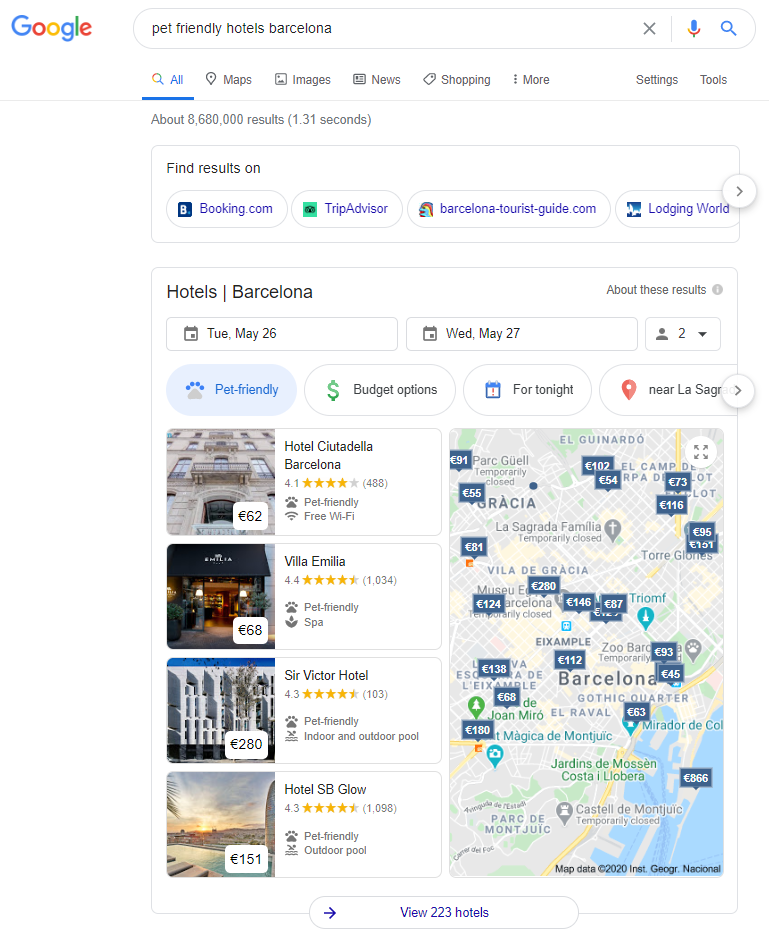A screenshot of Google search results for "pet-friendly hotels Barcelona." At the top of the image, the search query is visible in the Google search bar. Below, a map of Barcelona is displayed, showing several pet-friendly hotels highlighted with blue markers containing prices in euros per night. On the left side of the screen, there are four hotel options, each featuring a thumbnail image, a brief description, and user reviews that can be clicked on for more details.